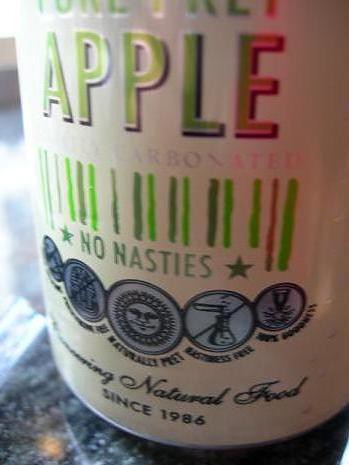This image showcases a closely-cropped view of a bottle, prominently featuring large green letters that spell out "Apple." Below this, in smaller silver letters, the word "Carbonated" is just barely visible. Further down, in green letters near what resembles a barcode, the phrase "No Nasties" is clearly written. The bottle also displays the phrase "Natural Food Since 1986." Additionally, there are five small round images, resembling medals, which likely highlight the beverage's features, such as what it does or does not contain.